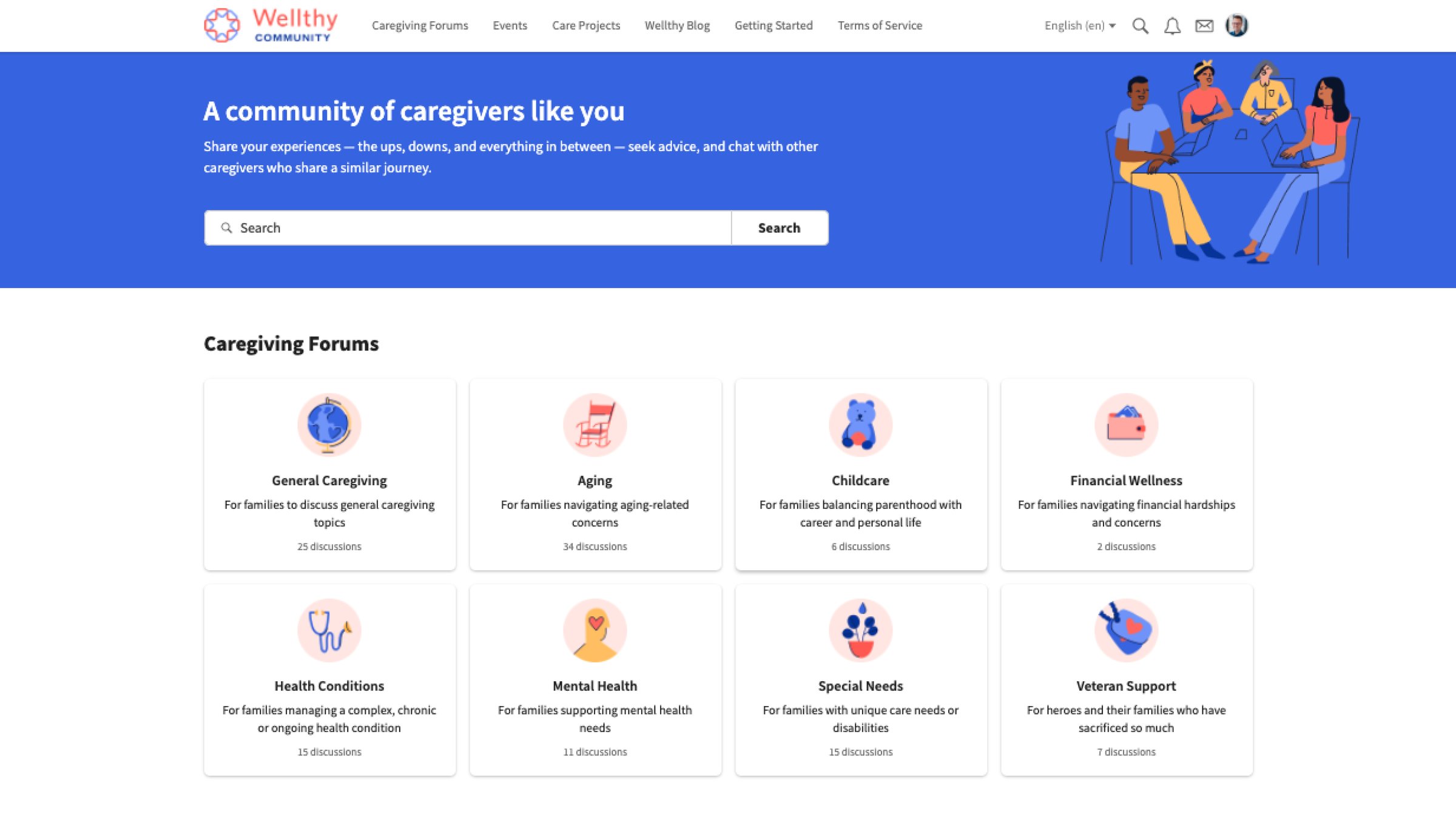In this vibrant and supportive online community, caregivers find a wellspring of resources and connections. The platform features comprehensive links to various caregiving forums, keeping members informed about upcoming events and ongoing care projects. Additionally, a richly informative blog offers a wealth of knowledge, helping caregivers to get started and understand the terms of service. Navigation is user-friendly with accessible options for searching content, receiving notifications, and sending messages. Each user has a dedicated page to personalize their experience. This community is designed for caregivers like you, providing a space to share your experiences—the highs, the lows, and everything in between. Here, you can seek advice and engage in meaningful chats with fellow caregivers navigating similar journeys. Specific forums are available for discussing general caregiving topics, as well as those related to aging and age-related concerns, ensuring that every family can find the support and information they need.